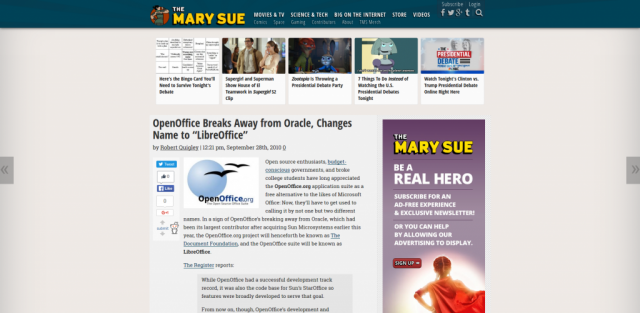The image features a gray rectangular background with a black rectangle at the very top. Inside the black rectangle, the name "Mary Sue" is prominently displayed in bold orange letters. Directly beneath this, there are five smaller squares arranged in a row. The details of the text beneath these squares are indistinct. 

- The second square contains a photograph of a man and a woman; she is dressed in a white sleeveless dress, and he is in a beige suit and tie.
- The content of the first and third squares is not visible.
- The fourth square displays a cartoon image of a young girl with short blonde hair, wearing a dress with puffy sleeves.
- The fifth square has an image that appears to be a person or cartoon, but it's too small to decipher clearly. There is some red and blue text crossing it.

Adjacent to these five squares on the leftmost side appears to be text-only, and a sequence of approximately ten small squares followed by a brief paragraph.

Beneath the row of five squares is a larger rectangle featuring text that promotes the use of LibreOffice, encouraging a transition from Oracle's OpenOffice. Next to this promotional text is an image of a full blue moon with either two birds or bats flying nearby.

On the far right of the gray rectangle is a call-to-action message from "The Mary Sue" encouraging users to become subscribers for a "real experience and exclusive newsletter" or to support by enabling advertisements. Below this message is a sign-up button.

Lastly, there's a cartoonish character shown from behind. This character has red hair and is wearing a red cape. Her arm, bent at the elbow, appears robotic or is outfitted with a red armband, though the small size makes the details hard to distinguish.